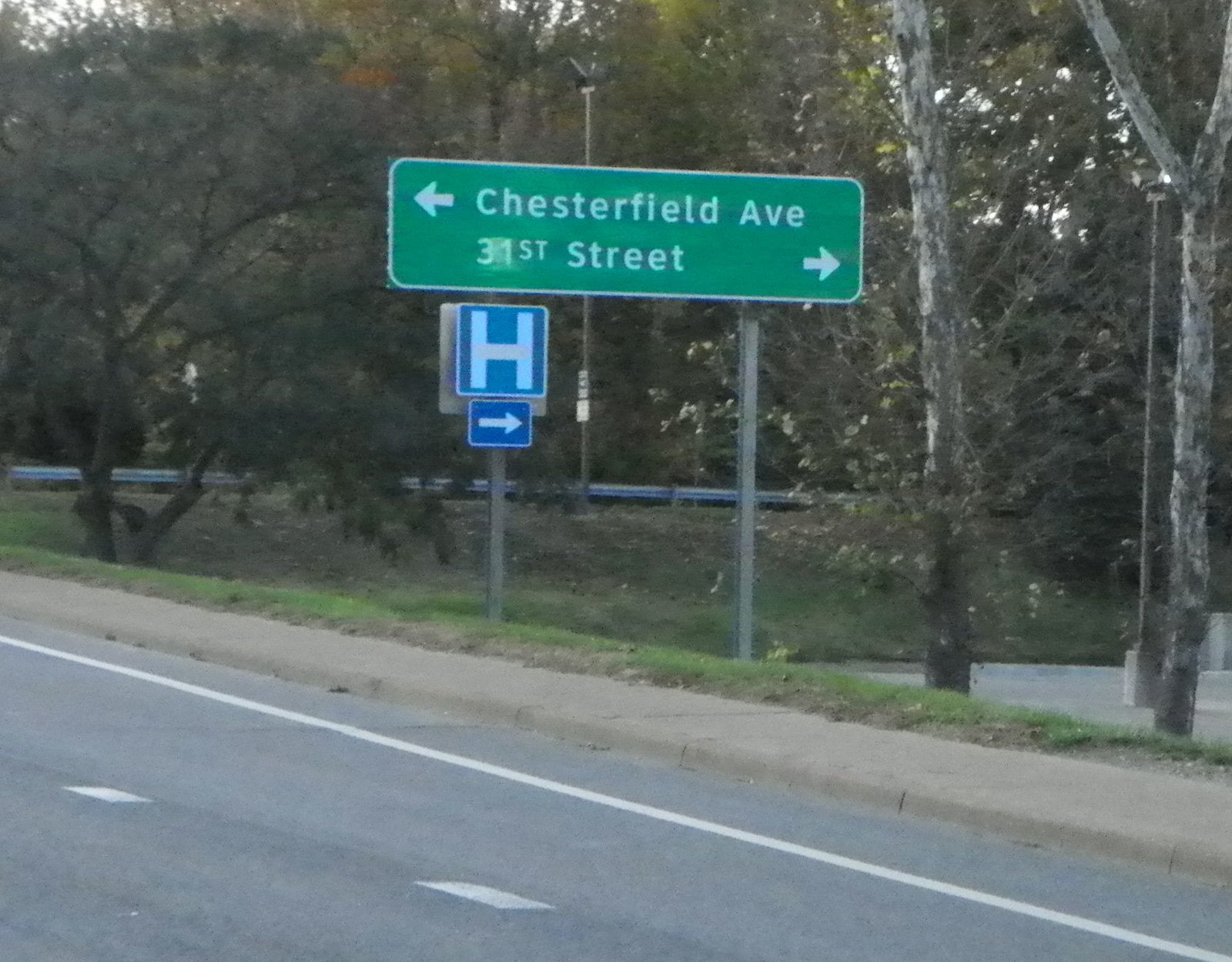In the image, we observe a road sign scene with detailed elements. At the bottom, a grey road with white dotted lines and a solid white line leads to a grey cement sidewalk. Behind the sidewalk, a small embankment covered in green grass is visible. Flanking the scene are numerous trees on both the left and right sides.

Prominently displayed in the middle are two grey poles. The first pole on the left features a blue sign with a large white "H" indicating a hospital, accompanied by a smaller blue sign below it with a white arrow pointing to the right. Adjacent to it, a green sign with white text and borders provides directional information: an arrow to the left indicating Chesterfield Avenue and an arrow to the right indicating 31st Street. In the background, a grey metal guardrail runs parallel to a lamp pole standing upright.